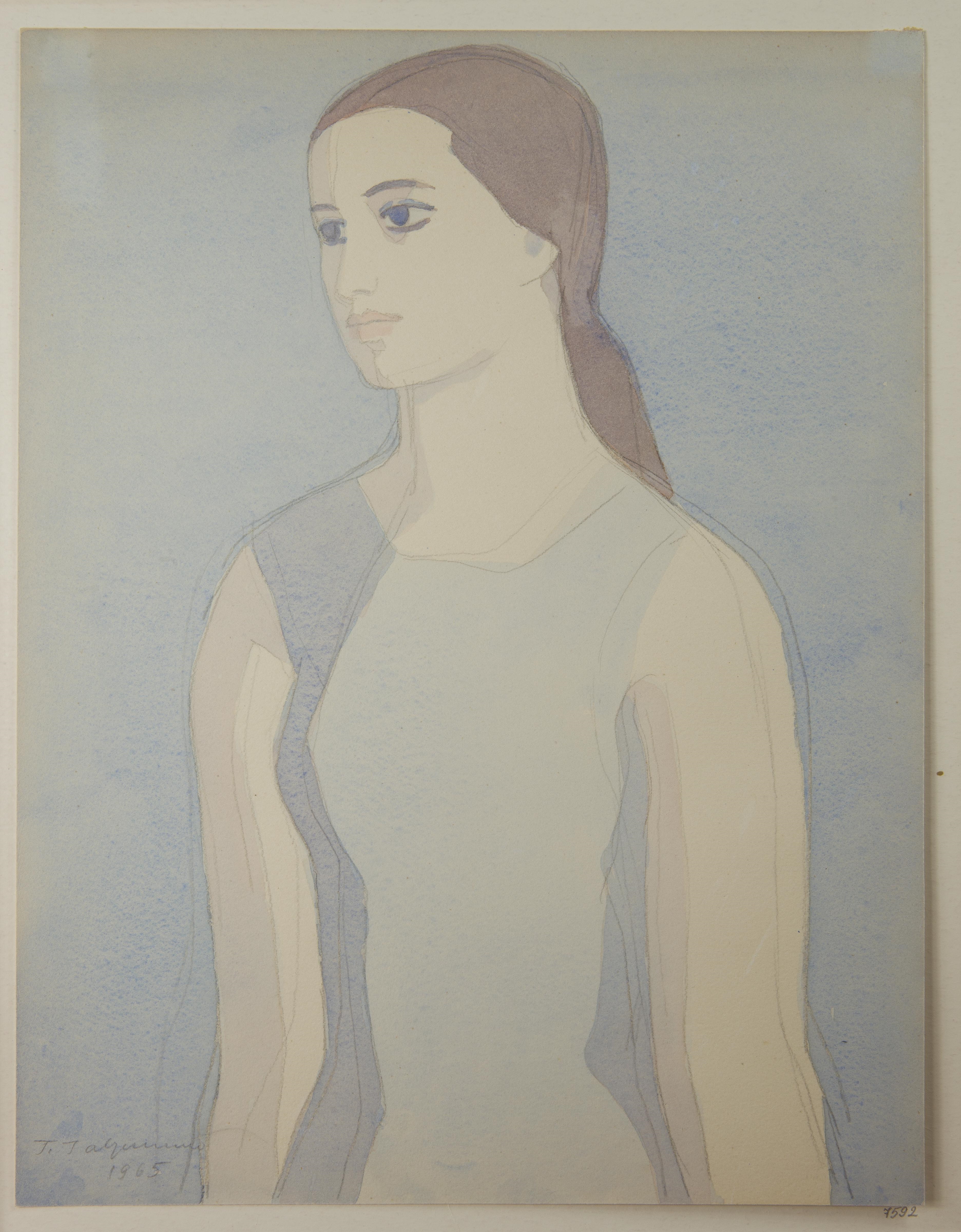This modern impressionist portrait, painted in watercolor or pastel, captures a woman in her mid-20s. The artwork is in portrait orientation, featuring the subject from the top of her head to her hips. The background is a gradient of sky blue, lighter on the left side and blending into a seamless wash toward a deeper blue on the right. 

The woman has long brown hair, flowing midway down her back, and is pulled back. She has blue eyes and brown eyebrows, her gaze directed to the left side of the image, complemented by a slight smile. Her complexion is fair, accentuated by pale, flesh-colored lips. 

She wears a sleeveless dress with thick straps and a square neckline, predominantly gray with hints of blue and dark gray accents. Her arms hang straight down at her sides, giving the impression she is standing still. The artist's signature and the date 1965 appear at the bottom left corner of the painting, though the name is not legible.